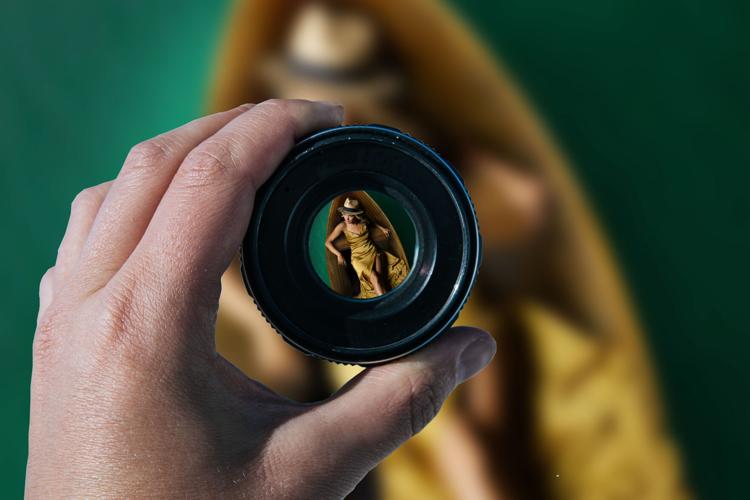This close-up photograph features a male hand, with unpainted fingernails, holding a black camera lens. Through the lens, a detailed reflection reveals a Caucasian woman with skinny arms and a light tan, lying down in a brown canoe on green water. She has blonde hair and is dressed in a golden short dress, complemented by a straw hat with a black band. The surrounding background is blurred in a green hue, making the focused reflection inside the lens the focal point of the image. The overall effect draws attention to the clarity within the lens against the blurred context of the woman in the canoe outside of it.